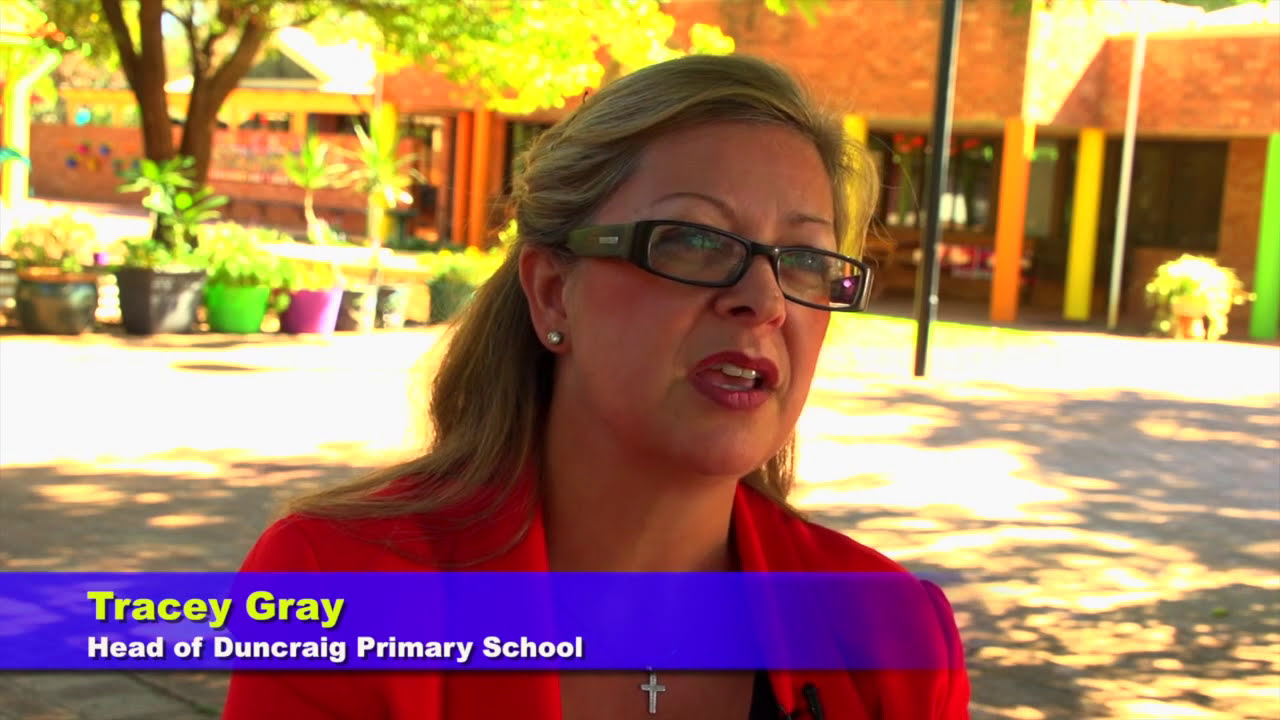The image captures a still frame from a news video featuring Tracy Gray, Head of Duncraig Primary School, who is being interviewed. Positioned centrally, Tracy Gray, a middle-aged woman with blonde hair tied back in a ponytail falling to her shoulders, wears a bright red blazer, complementing her black-framed prescription glasses. Her noticeable accessories include a silver cross necklace and a small diamond stud earring in her right ear. Tracy's mouth is open, indicating she is speaking, and a small black microphone is clipped to her blazer. At the bottom of the screen, a blue rectangular banner with the text "Tracy Gray" in off-yellow font and "Head of Duncraig Primary School" in white font is displayed. The backdrop reveals a large brick school building with sizable windows and doors. The scene also includes potted plants and a leafy tree with sunshine casting shadows on a walkway behind her. The setting suggests the vibrant and welcoming environment of the primary school.